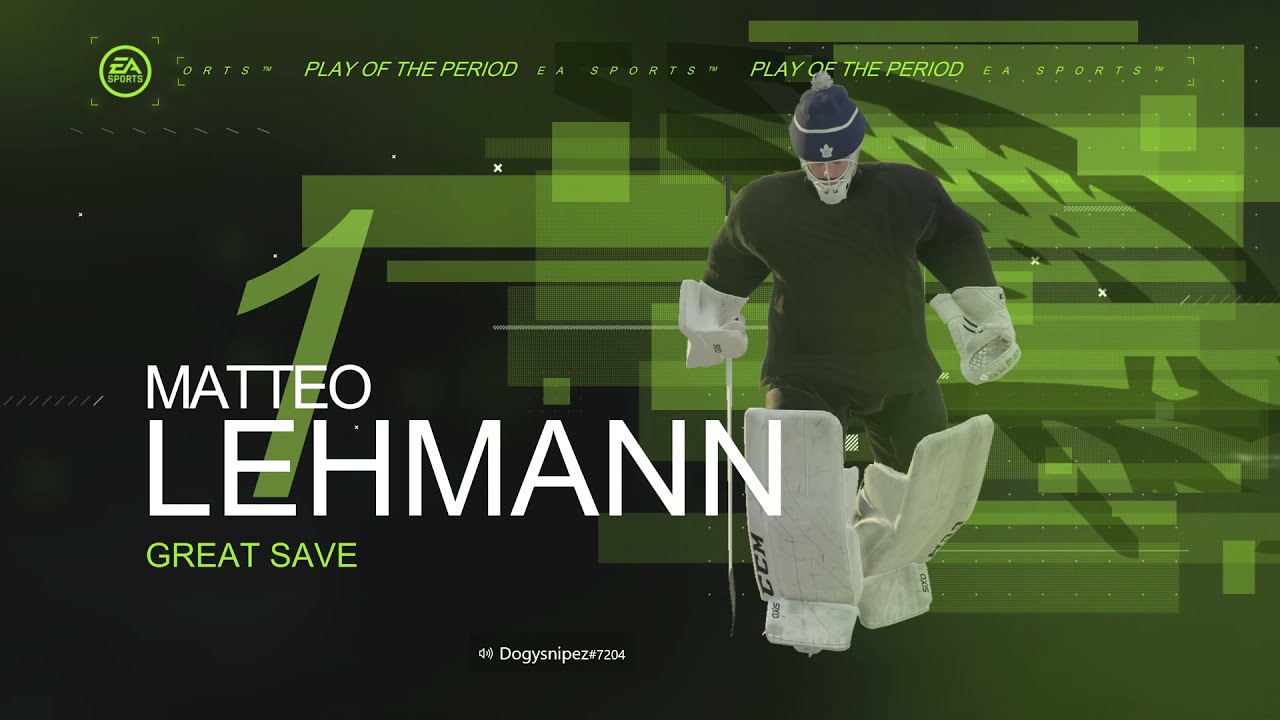The image is a detailed screenshot from a hockey video game by EA Sports. In the top left corner, there’s a green EA Sports logo with text that reads "Play of the Period." The central focus is a hockey player, a goalie named Matteo Lehmann, who is prominently featured with his name spelled out clearly. Lehmann is dressed in a solid dark green outfit with white padding on his legs and hands, a white face mask, and he’s topped with a blue cap. The player's number, "1," is displayed in green behind his name. Beneath the name Matteo Lehmann, green text reads "Great Save." The background behind Lehmann is a futuristic, cyberpunk-style combination of black and green with abstract squares and rectangles, giving it a cool, modern appearance. Additionally, towards the bottom, there is text that says "Dougie Snipes" alongside a speaker symbol, indicating that someone is speaking while playing the game. The overall impression is sleek and dynamic, emphasizing Lehmann's significant in-game moment.